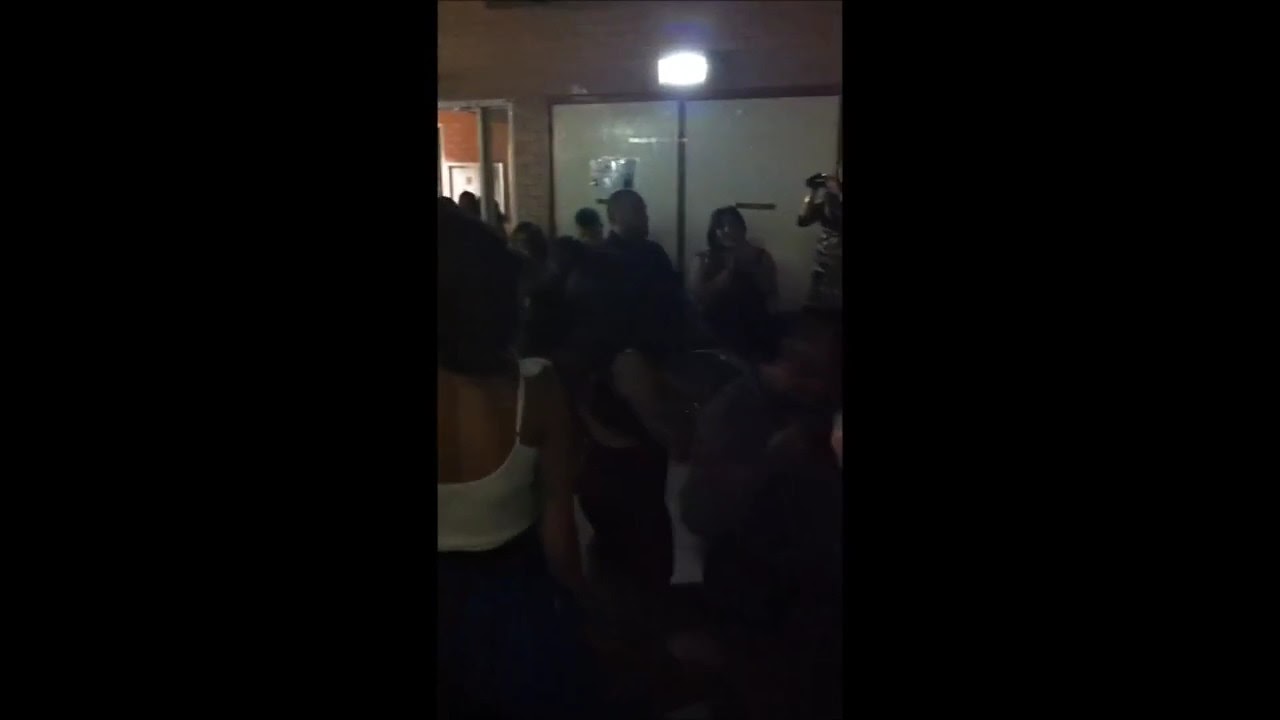In this dimly lit indoor gathering, a diverse group of men and women are milling about a room with noticeable brick walls and dark ambiance. A soft white fluorescent light on the ceiling attempts to illuminate the scene, casting shadows that highlight the dinginess of the space. Closest to the viewer is a brown-skinned woman dressed in a white top that exposes her back and a black bottom. Beside her, another woman similarly attired in black, her hair dark and cascading. Near an open doorway at the far left of the image, which is bright with light, stands a man with a shaved head and short hair. Above this doorway, a whiteboard with a framed laminated paper is visible. The room also contains window panes with brown frames, although their shutters obscure any outside view. This gathering seems casual, with the attendees engaging in low-key conversations, their faces mostly turned away or obscured by shadows. The overall mood suggested by the photograph is muted and intimate, hinting at a quiet social interaction amidst the dim surroundings.